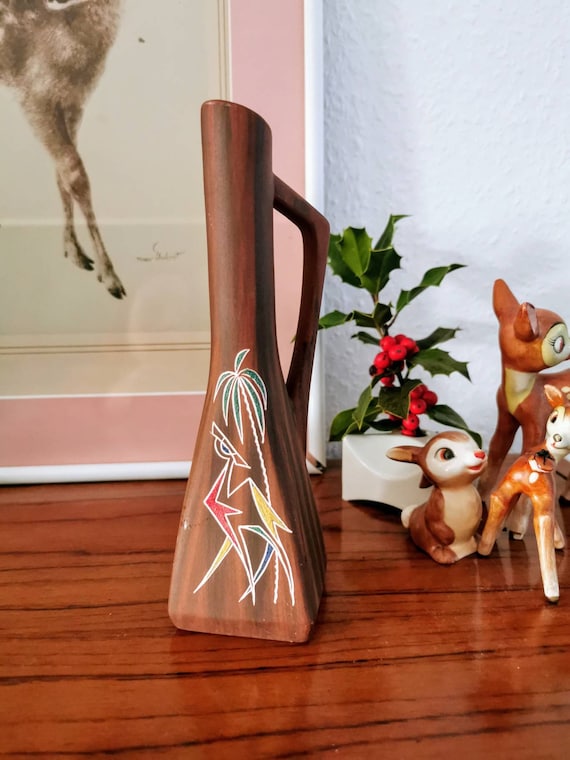The close-up photo features a tall, slim wooden cup with a handle, resembling a vase or bottle, adorned with a design of a tree with a long thin white trunk, six green leaves, and an abstract animal painted in bright colors—red, yellow, transparent, green, and blue. This object is resting on a shiny dark maple wood floor. Surrounding the wooden cup are small figurines, including deer and a rabbit. To the side, there is a faux plant with green leaves and red berries, likely representing holly. In the background, a framed photo with a pink border and a white frame is visible, showing partial imagery of an animal with two legs and part of the torso; the frame leans against a white, textured wall. The overall scene features a palette of brown, yellow, red, blue, green, and white, with hints of pink, capturing a rustic and festive atmosphere.